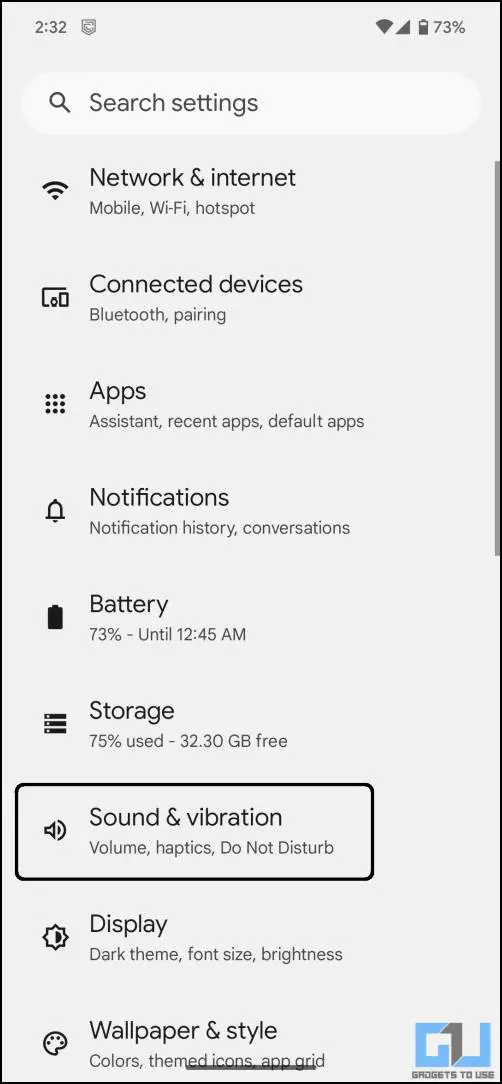This image is a screenshot of a mobile application interface featuring a light gray background that runs vertically along the entire height of the page. At the very top is a pale gray search bar with an elongated pill shape, containing a medium gray magnifying glass icon on the left and medium gray text reading "Search settings" to its right. 

Below the search bar, there are several rows of information, each row featuring a dark gray icon on the left and large gray text on top with smaller light gray text beneath it on the right. 

The list of icons and corresponding information from top to bottom includes:
 
1. A Wi-Fi icon linked to "Network & internet" with the subtext "Mobile Wi-Fi hotspot."
2. An icon showing multiple electronic devices representing "Connected devices" with "Bluetooth pairing" as the subtext.
3. A grid of nine dots indicating "Apps" with "Assistant, recent apps, default apps" as the detailed view.
4. A bell icon for "Notifications," elaborated with "Notification history, conversations."
5. A fully charged battery icon marking "Battery" with detailed info "73% – until 12:45 AM."
6. Three stacked rectangles symbolizing "Storage," detailing "75% used – 32.30 GB free."
7. A volume icon representing "Sound & vibration" which includes further details "Volume, haptics, do not disturb."

These rows of information are encased within a black rectangle outline with rounded corners, with more information rows extending beneath this outlined section.